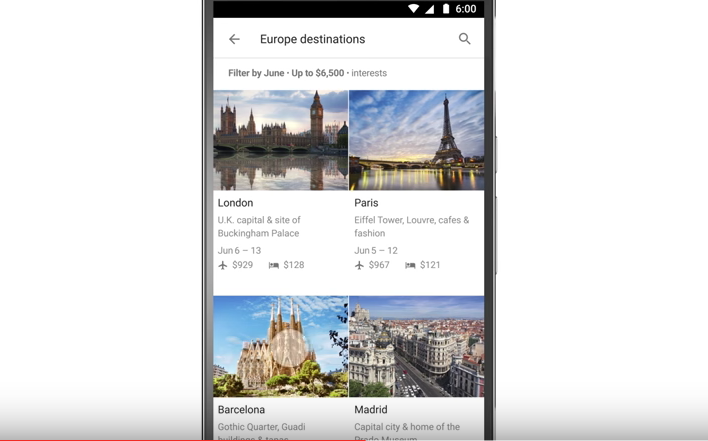The image is a detailed mock-up of a cell phone display on a website. At the very bottom of the screen, there is a gradient transitioning from white to gray, along with a red progress bar that spans halfway across the screen, indicating loading or playback status.

The primary image displays a cell phone with visible side buttons and a slightly reflective metal on the left edge. The top portion of the cell phone extends beyond the visible frame, creating an incomplete view. At the top of the cell phone screen, status icons show Wi-Fi connectivity, full battery, and signal strength, along with a time display reading 6:00.

The header of the cell phone screen includes navigation elements: a back arrow, a magnifying glass for search, and the text "Europe Destinations." Below the header, promotional information states, "Hold it by June, up to $6,500," along with an "Interest" section showcasing travel deals to various European cities with accompanying photographs.

The first section features details about London, showcasing an image of Big Ben and reflective lights along the Thames River. The travel package reads: "London, UK Capital inside of Buckingham Palace," dated June 6th to 13th, priced at $929 for airfare and $128 for accommodations (indicated by a bed icon).

Next, Paris is highlighted with images of the Eiffel Tower and the Louvre. The package includes: "Paris, Eiffel Tower, Louvre, Café and Fashions," dated June 5th to 12th, priced at $967 for airfare and $121 for accommodations.

Below these, there are mentions of additional destinations like Barcelona, noted for Gothic Gaudí architecture and a cathedral, with details partially obscured. Similarly, Madrid is included, described as the "capital city and home of the..." with the rest of the text cut off, likely referring to a significant cultural site such as the Prado Museum.

Overall, the image serves as a visual guide for a travel booking website, offering detailed and visually appealing previews of travel packages to European destinations.